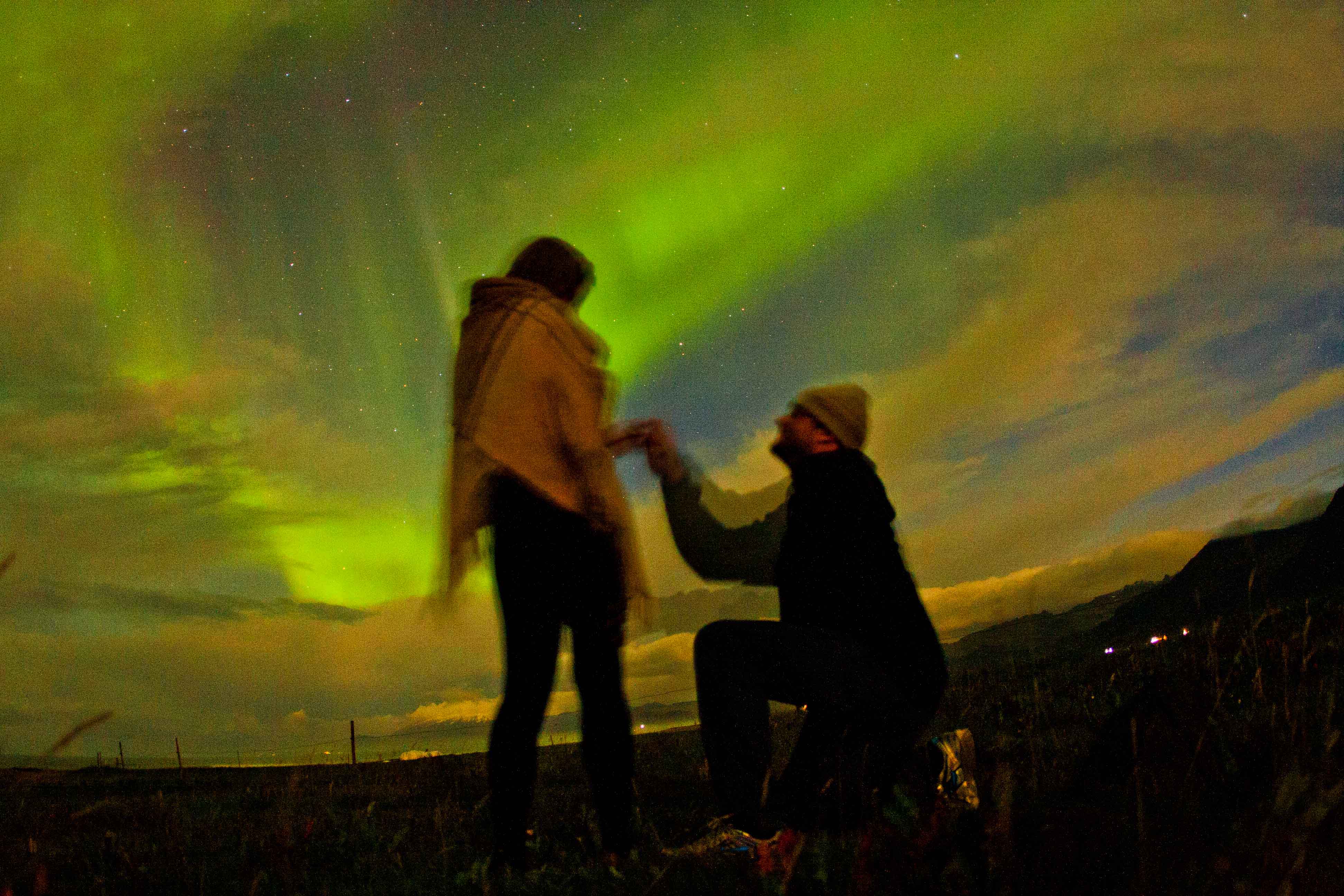In this captivating painting, a man is down on one knee proposing to a woman in a dark, grassy field with some overgrown patches of green and tan grass. His right hand tenderly holds her left hand as he looks up at her. The man is dressed in a dark-colored outfit and sports a tan beanie, while the woman is adorned in a light tan shawl and black pants. The romantic scene is set against an enchanting evening sky, predominantly dark with cloud coverage, yet revealing streaks of the mesmerizing Aurora Borealis. Green and purple hues from the aurora dance across the sky, alongside a fading blue twilight. In the background, on the bottom right, subtle mountainy hills add depth to the landscape. The composition, which appears to be viewed from ground level, beautifully captures the essence of the intimate moment under the vast, celestial spectacle.